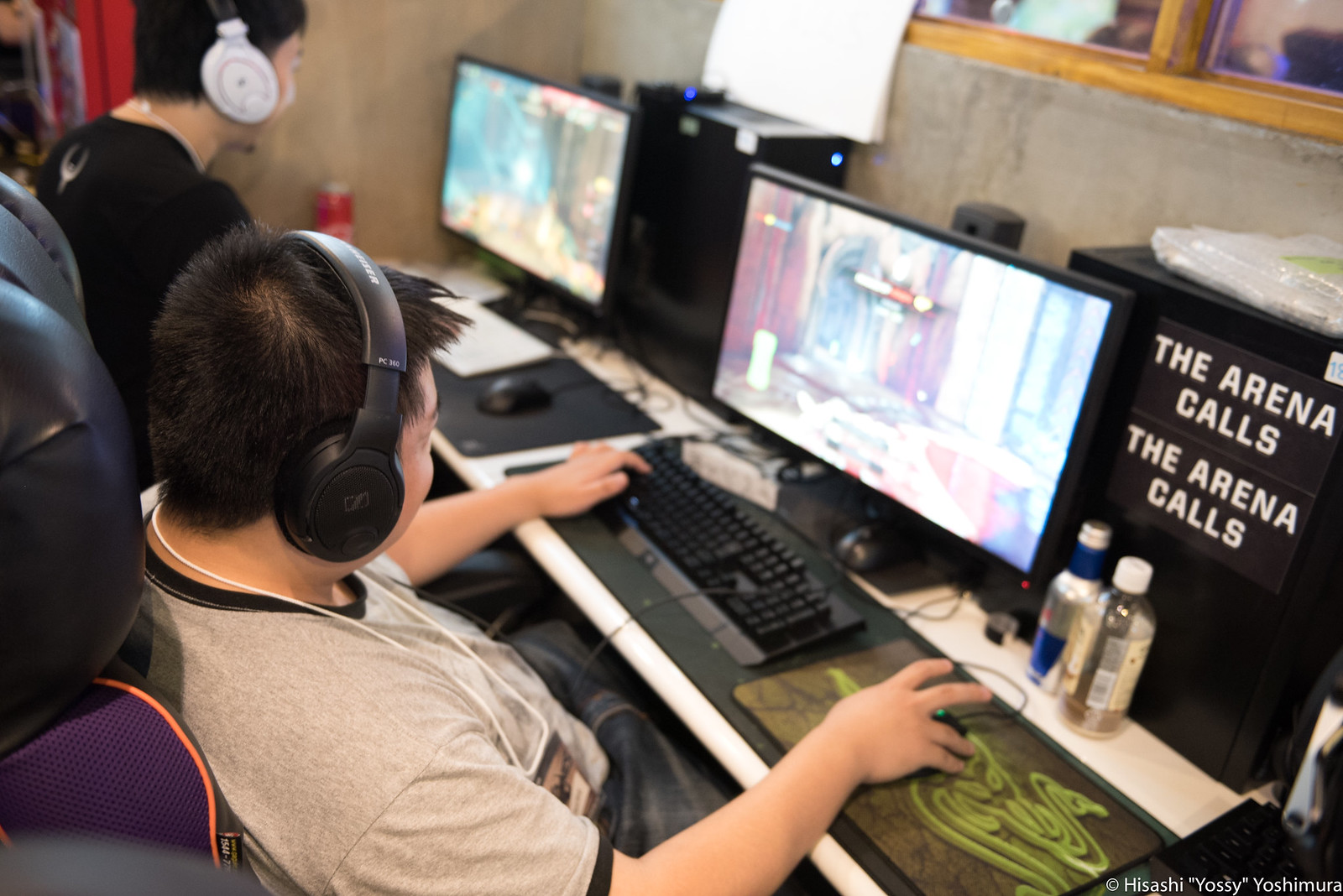The image depicts two men engrossed in playing video games at a desk, viewed from a side and back angle. Both men are seated in black computer chairs with leather upholstery. The man on the left, further from the camera, wears a black T-shirt and white over-the-ear headphones, and he has black hair. He is focused on his computer screen, which appears to display a video game, possibly a first-person shooter. 

The man closer to the camera is dressed in a gray T-shirt with black trim on the cuffs and collar. He also has black hair and is wearing black over-the-ear headphones. His left hand rests on the keyboard while his right hand maneuvers the mouse, indicating active gameplay. Both men are using large, widescreen monitors. 

On the desk, there is a prominent sign with a black background and white text that reads "The arena calls," repeated twice. Nearby, computer towers in sleek black cases are positioned behind their monitors. The player closer to the camera also has a mouse pad featuring the logo of the gaming brand Razer. Additionally, two bottles are placed to his right, with one appearing to be water. The setting includes gray cement walls and a window above the computers with a light brown wooden frame, suggesting an industrial or minimalist space, possibly a LAN center.